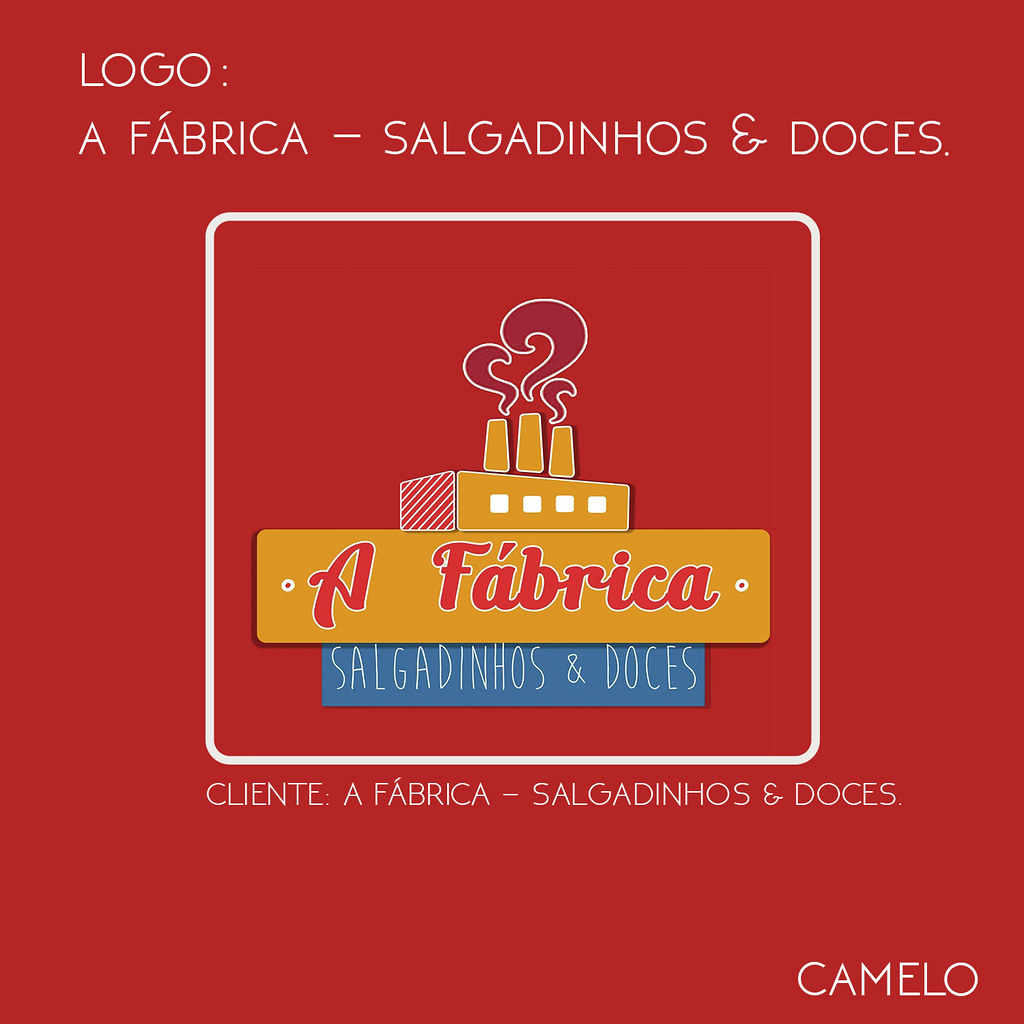This image is a detailed graphic banner, designed with a combination of illustration, typography, and graphic design, and formatted in a square layout. The background is a solid red color with prominent white text at the top that reads: "LOGO: A.FABRICA-SALGADINOS & DOSIS." Below this, there is a white-outlined square with curved corners containing an illustration of a factory in a gold color, emitting swirls of red from three exhaust towers. Directly beneath the factory illustration, there is a horizontal gold sign with red script lettering that says "A. FABRICA." Underneath this sign, another horizontal stripe features the white text: "SALGADINOS & DOSIS."

Further down, outside the white square, another line of white text reads: "CLIENT: A. FABRICA-SALGADINOS & DOSIS." In the bottom right corner of the banner, the word "CAMELO" appears in white text. The entire design utilizes both illustrative and typographic elements to create a visually cohesive graphic, and it appears to be in a foreign language.